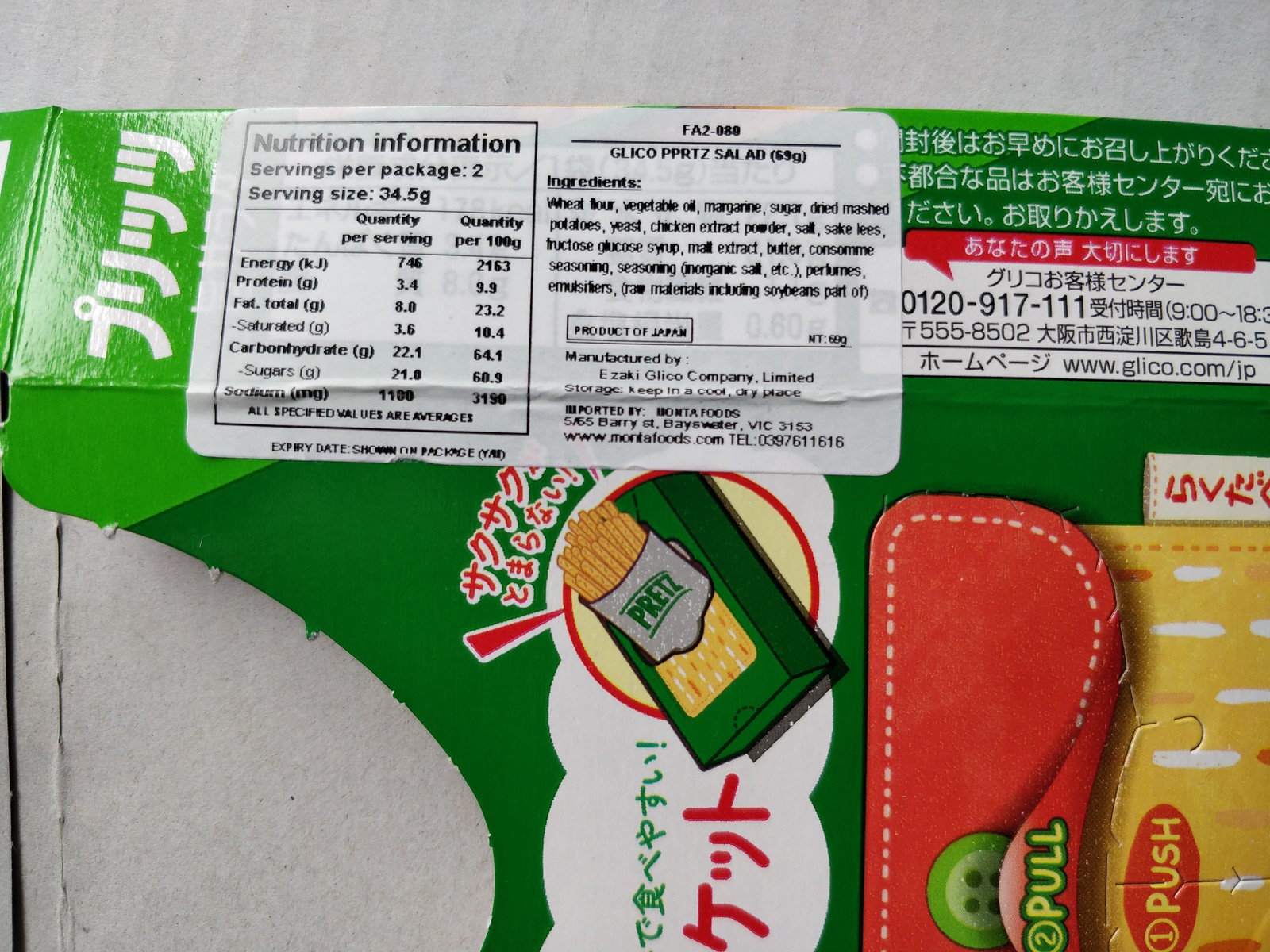This close-up photograph captures the detailed label of a rectangular-shaped, chip-like snack from Glico, known as Pretz. The packaging is primarily dark green with an orange and white rectangular pattern on the background. It features a gray bag with white dots and dark green diagonal lines at the top and bottom, displaying the word "Prez," P-R-E-T-Z. The snack inside the packaging is depicted as dark brown fries with spots. The label also includes a nutrition facts section specifying serving size as 34.5 grams per serving, with two servings per package. The nutritional values listed are energy 746/2163 (assumed to be kcal per serving/total), protein 3.4 grams/9.9 grams, total fat 8.0 grams/23.2 grams, saturated fat 3.6 grams/10.4 grams, carbohydrates 22.1 grams/64.1 grams, sugars 21.8 grams/68.9 grams, and sodium 1100 mg/3190 mg. Additionally, there's a white rectangle on the right side displaying the contact number 0120-917-111 and the website www.glico.com/UK. The packaging is green overall and includes a pull and push mechanism, highlighted with “Pull” in green and “Push” in red. It also features Japanese text and instructional imagery on how to open and use the box, aligned with red and yellow perforations.